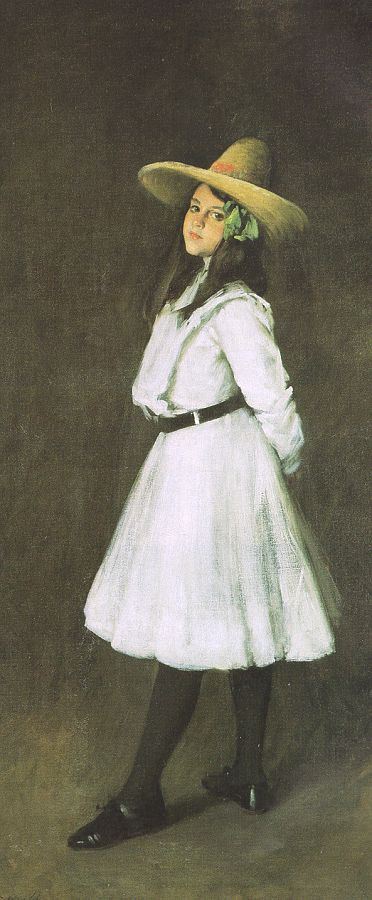The image depicts an incredibly realistic oil painting of a young girl standing against a dark background, which appears to be a blend of brown, grey, and dark olive hues. The girl's stance shows her body facing left, with her left foot pointing towards the bottom left corner and her right foot pointing to the wall, while her face is turned towards the front, almost engaging the viewer with a blank, contemplative stare. She is dressed in a white, knee-length dress with long sleeves that reach her wrists, cinched at the waist by a black belt featuring a grey buckle in the front. Her legs are adorned with black stockings, and she wears black, closed, flat shoes. Perched on her head is a tall straw hat with a pointed dome and a slightly bent brim towards the back, adorned with a small orange spot and some green flowers or a cloth bow on the left side. Her dark brown, almost black hair, frames her small nose and little lips, complementing her dark eyes. The intricacy of her attire and the somber yet captivating background enhance the painting’s realistic and detailed nature.